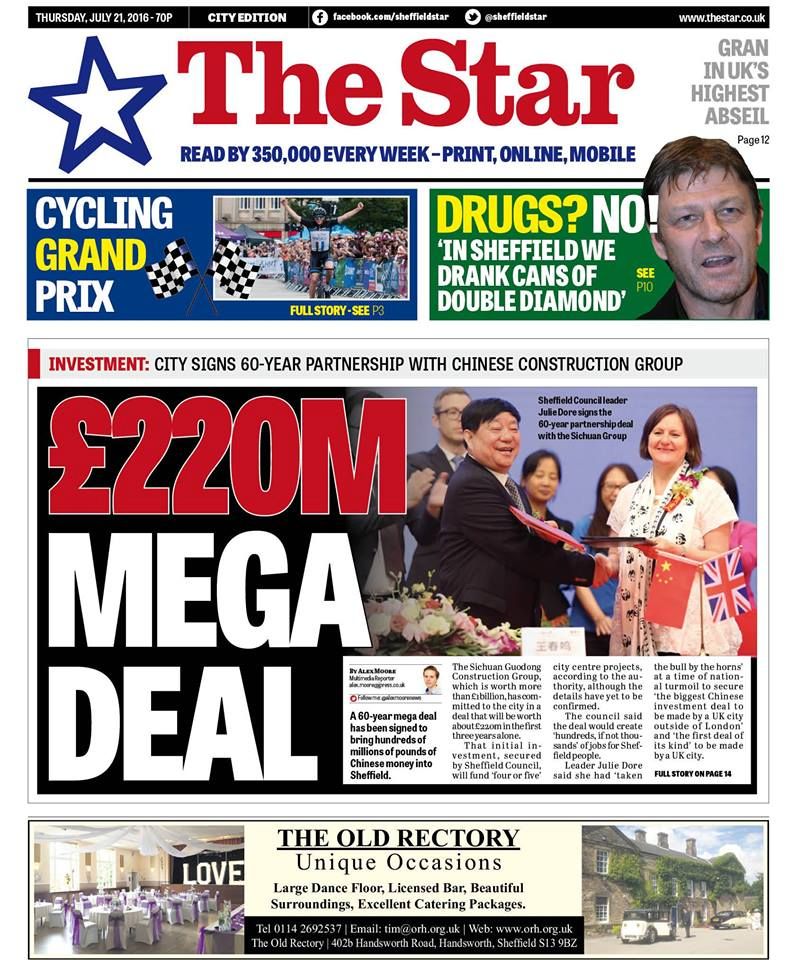This image is a screenshot from the tabloid magazine, *The Star*. The top banner displays the publication date as Thursday, July 21st, 2016, with a price of 70p, labeled as the city edition. Social media icons present indicate links to Facebook and Twitter, though the Facebook link is too small to discern clearly.

At the center, a prominent blue star features the title *The Star* in red lettering. A tagline reads, "Read by 350,000 every week," with further distribution methods listed as print, online, and mobile.

Beneath the title, two distinct stories are highlighted. On the left, there is a headline for the "Cycling Grand Prix," accompanied by an image of a cyclist racing past a cheering crowd, with an interactive option to click for the full story. On the right, another headline states, "Drugs? No, in Sheffield we drank cans of Double Diamond," paired with a picture of actor Sean Bean.

Further down, the segment labeled "Investment" announces, "CitiSign 60-year partnership with Chinese Construction Group, 220 million mega deal." Below the headline is a brief excerpt of the story and an image depicting a man and a woman shaking hands.

The bottom section appears as an advertisement for *The Old Rectory*, listing features such as a large dance floor, licensed bar, beautiful surroundings, and excellent catering packages. Contact details, including an email address and phone number, are noted, flanked by additional images on both sides.